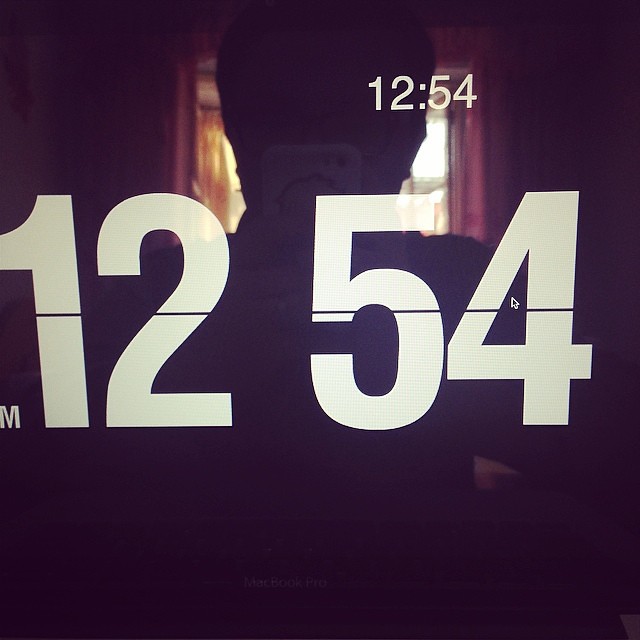This image is an indoor, extreme close-up photograph of a digital clock displaying the time "12:54" in large white font across the center, with a line through the middle of the numbers. In the upper portion of the image, slightly right of center, the time "12:54" is repeated in a smaller white font. The photograph is dark, with the lower third of the image almost completely black. The major feature of the image is the reflection of a person taking a selfie with their smartphone. The person, whose face and clothes are obscured by the darkness, is holding a phone with a white case in their right hand. They appear to be facing forward and may be wearing glasses. Behind the person is a window with pinkish-purple curtains on the right and yellow-orange curtains on the left, casting light that helps create their silhouette. A part of the reflector, likely a mirror or a screen, is visible at the bottom edge of the photograph.